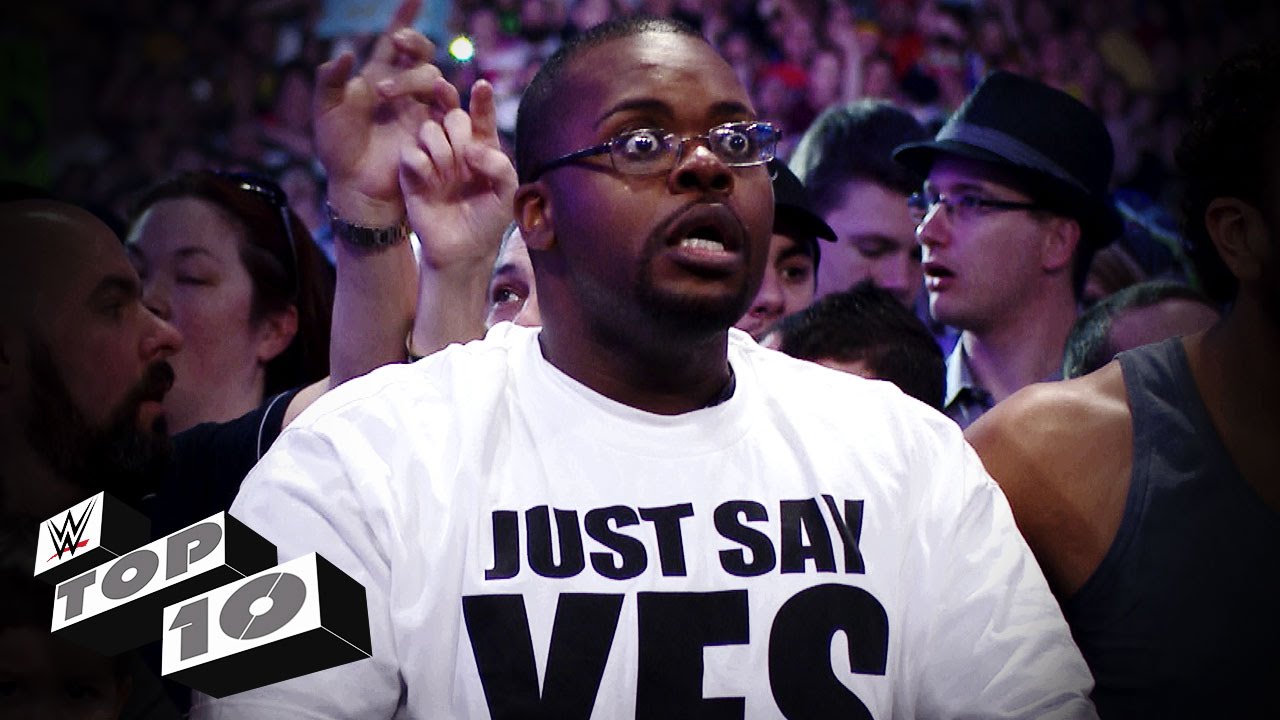The photograph captures an energetic moment at a World Wrestling Entertainment (WWE) event. Dominating the center of the image is a large man wearing a white T-shirt with bold black lettering that reads, "Just Say Yes," though the word "Yes" is partially cut off at the bottom. He has short black hair, glasses, and his mouth is open wide in surprise, which is accentuated by his bugged-out eyes. The excitement on his face is a focal point, enhanced by the vivid detail of his open mouth showing his bottom teeth. 

In the background, a lively crowd elevates the atmosphere, with people gesturing energetically—some with hands raised, one even wearing a watch. To the left of the central figure, there are items featuring the WWE logo, “Top Ten,” and a prominent “W.” Over his shoulder, various attendees can be seen; a man and a woman are distinctly visible to the left, while a man in a hat and glasses is noticeable on the right. The broader crowd fades slightly out of focus, suggesting a dynamic and bustling event. The blend of the central figure's exaggerated expression and the bustling crowd behind him vividly conveys the high-energy atmosphere of the WWE event.